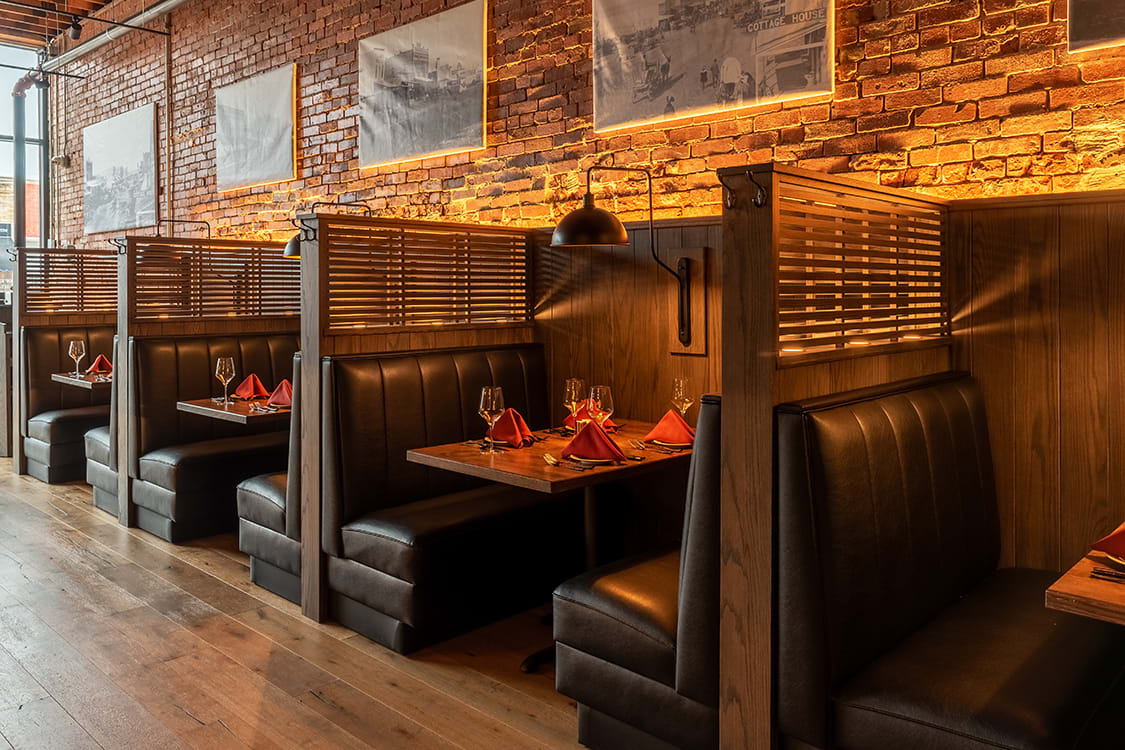The image captures the interior of a well-lit restaurant, prominently displaying four booths in a row against a red brick wall. Each booth features high-back benches padded in a black finish with slotted wooden panels on the sides, providing a touch of privacy. Between each booth, vertical wood planks serve as natural dividers. Above each booth, old-time framed pictures add a nostalgic charm. Hanging over each booth is a round, half-circle light, ensuring that each seating area is well illuminated.

The booths, tables, and the floor all share a rustic wooden aesthetic, creating a warm and cohesive environment. Each wooden table is neatly set with folded red napkins on plates, silverware on both sides, and uniform wine glasses poised at the end. Additionally, there are hooks on the outer wooden panels for hanging coats, illustrating attention to detail in guest convenience.